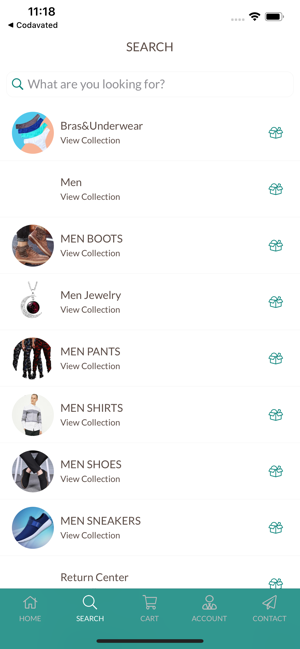Screenshot of a Minimalist Shopping Website

The screenshot displays a clean and simplistic design of a shopping site, likely viewed on a tablet. The entire background is white, providing a stark contrast to the black text, which improves readability. The layout is notably minimal, lacking fancy graphics or vibrant colors.

In the top left corner, the time is shown as "11:18" in black print. Directly beneath it is text that reads "Code updated," accompanied by a left arrow indicating a back navigation option. At the top center of the screen is a search bar, inviting users with the prompt "What are you looking for?"

Below the search bar, there is a linear arrangement of various clothing categories, each represented by a small oval icon on the left except for one:

1. **Bras and Underwear**
   - Icon Present
   - "View Collection" option

2. **Men**
   - Icon Missing
   - "View Collection" option (This collection likely serves as an umbrella category.)

3. **Men Boots**
   - Icon Present
   - "View Collection" option

4. **Men Jewelry**
   - Icon Present
   - "View Collection" option

5. **Men Pants**
   - Icon Present
   - "View Collection" option

6. **Men Shorts**
   - Icon Present
   - "View Collection" option

7. **Men Shoes**
   - Icon Present
   - "View Collection" option

8. **Men Sneakers**
   - Icon Present
   - "View Collection" option

Each clothing item listed has a small, clickable icon on the far right side of the screen, resembling a small box.

At the very bottom of the screen, a medium bluish-gray bar contains navigation tabs in white text: "Home," "Search," "Cart," "Account," and "Contact." The "Search" tab is highlighted, indicating that the user is currently on the search screen.